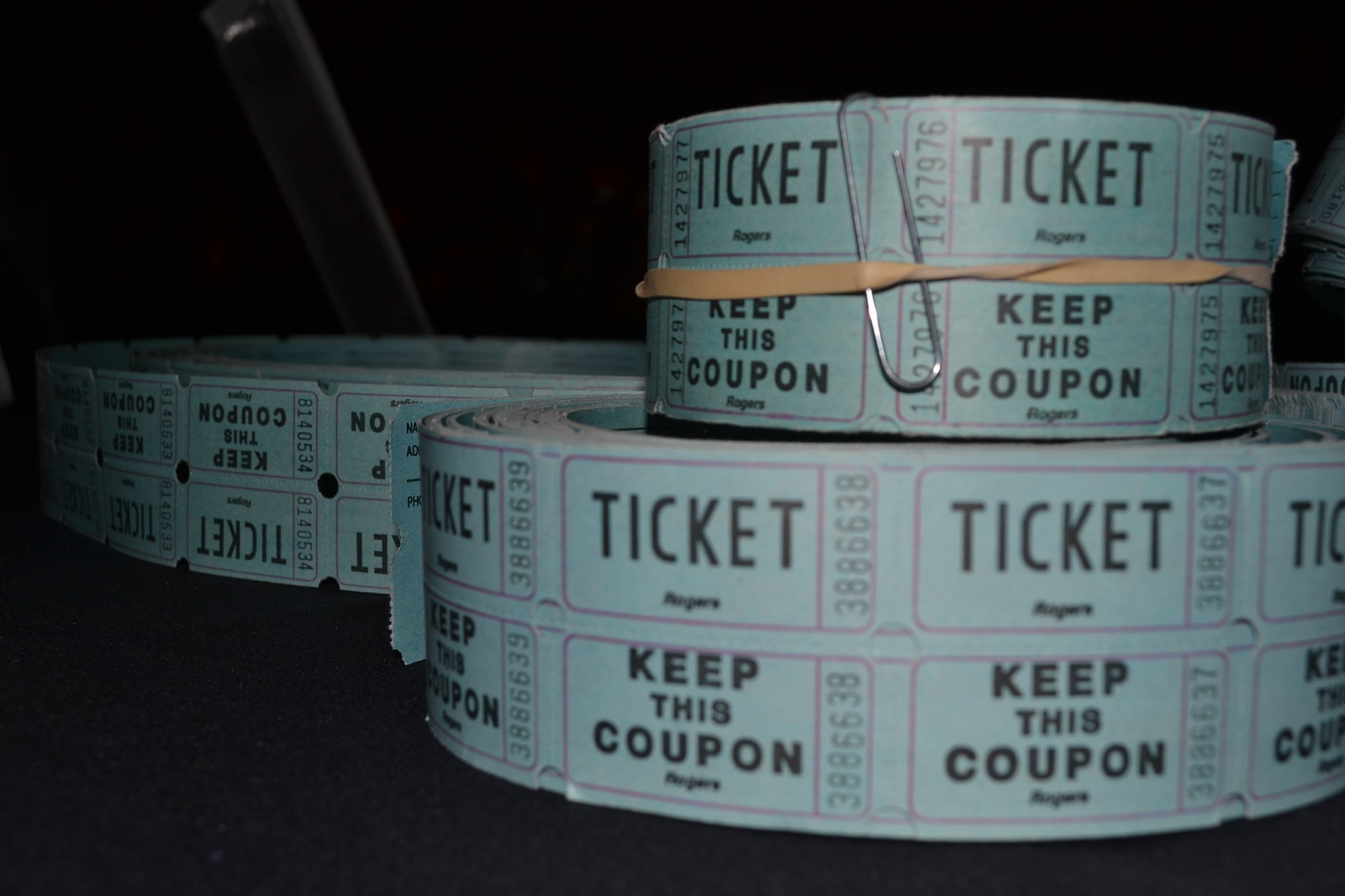In the dimly lit image, four rolls of aqua blue raffle or movie tickets are prominently displayed on what appears to be a dark fabric surface, potentially carpet or a car seat. The tickets, encircled by a rubber band and a paperclip, feature the text "Ticket, keep this coupon" at the top. One of the ticket rolls has the number 3886638, suggesting they follow a sequential order. The tickets, which range in size with some smaller rolls positioned above the larger ones, are centrally placed with one roll notably upside down. The background remains indistinct, emphasizing the vivid blue of the tickets against the predominantly black environment.